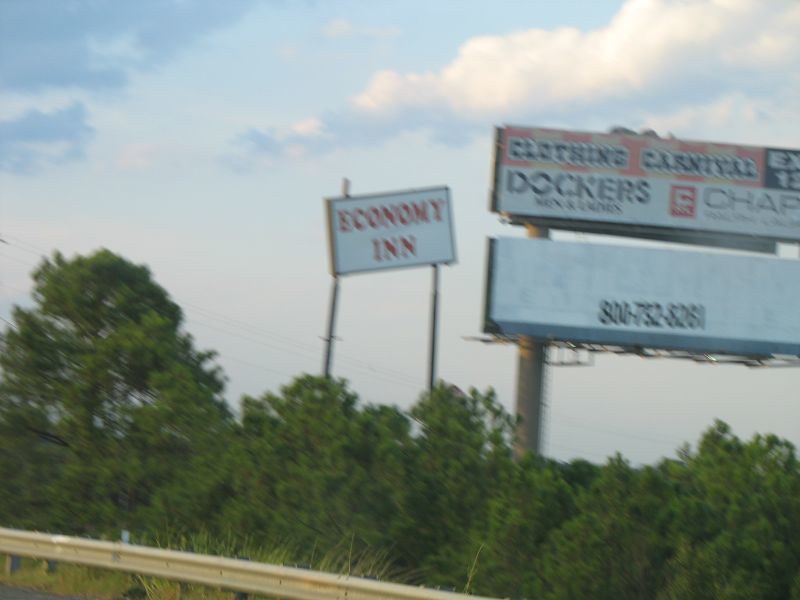The photo captures a roadside scene taken from what appears to be a moving car, causing some blurriness and graininess. Dominating the foreground is a metal guardrail along the edge of the road, behind which lies a steep embankment covered with high grass. Beyond the grass, tall green trees with thick, dark green leaves create a natural backdrop. Rising above the trees are two rectangular billboards stacked one on top of the other. The bottom billboard features a blank white space with black numbering advertising the number 800-752-8261 for potential buyers of the advertising space. Directly above it, another billboard promotes a "Clothing Carnival" with brands like Dockers and Chaps. To the left of these billboards, another sign supported by two metal poles and slightly crooked, announces the "Economy Inn" in red text on a white background. The sky overhead is a light blue with fluffy white clouds scattered about, indicating a sunny day.